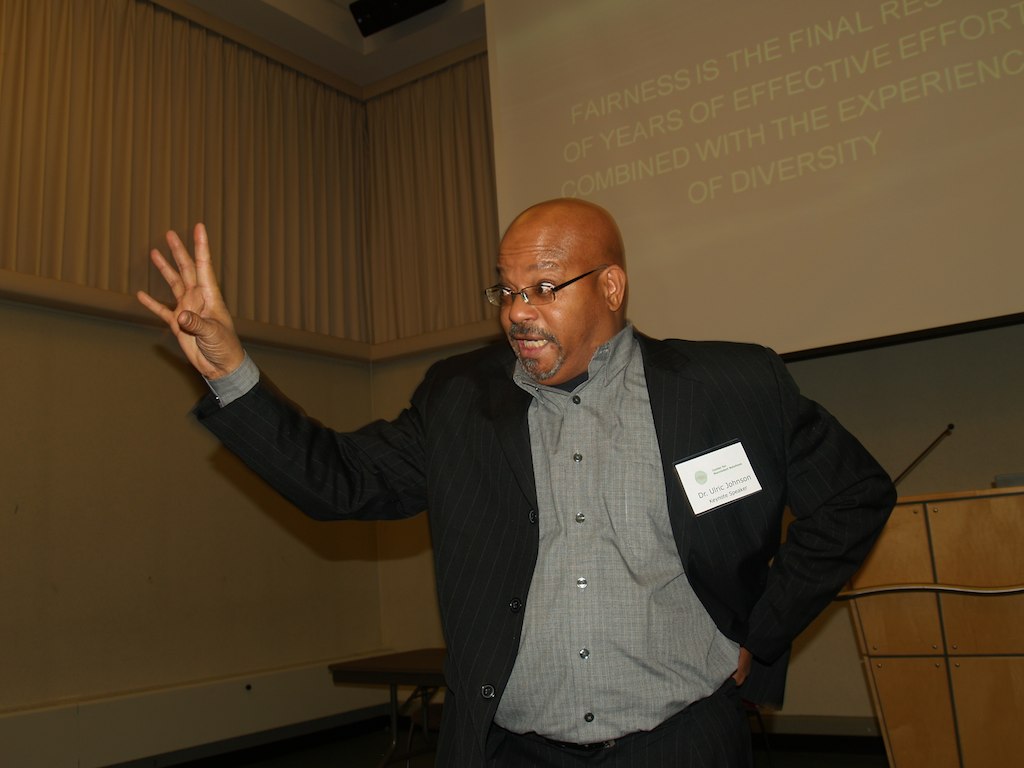The photograph depicts an African American man, bald with a gray goatee and wearing black-framed reading glasses, standing at the center of a room, gesturing with his right hand raised and all fingers extended. He is dressed in an open, dark blazer with gray pinstripes, paired with a gray button-up shirt featuring a light square pattern. A white name card is pinned to the left breast of his blazer, partly visible, reading "Doctor Johnson." The man is positioned slightly facing left of the camera and appears to be speaking to an off-camera audience, with an earnest expression on his face.

In the background, there is a large projection screen displaying partially cropped text that reads: "Fairness is the final... of years of effective effort... combined with the experience... of diversity." The background also features a light brown wooden podium, with a black microphone stand but no microphone attached. The man casts a noticeable shadow on the cream-colored wall behind him due to the projection screen’s light. At the upper left corner of the room, there are pleated curtains which seem to be designed for acoustical purposes. Additionally, to his left, a small desk with a wooden top and gray metal bottom and a metal chair are visible, accentuating the room's professional setting.